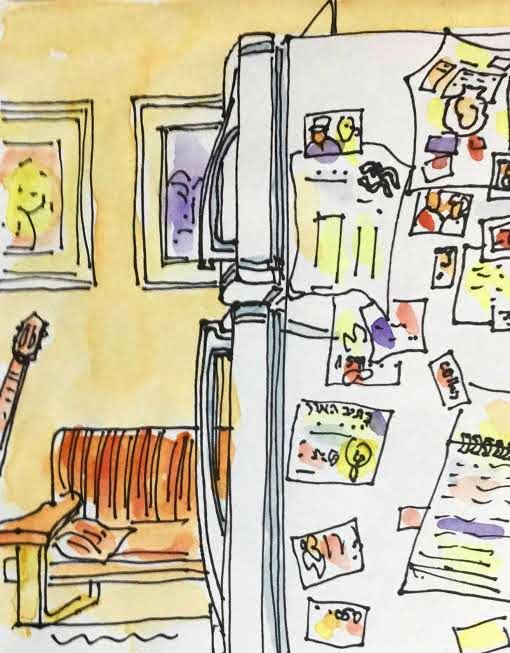The image is a cartoon-style watercolor drawing depicting a cozy kitchen scene. Dominating the right side of the composition is a large white refrigerator adorned with a variety of items held in place by magnets, including pictures, drawings, and papers. The refrigerator occupies nearly half of the page. In the background, the walls are painted a warm, yellow hue, adding to the room's inviting atmosphere. There are two vibrant paintings hanging on this yellow wall; one mainly features yellow and peach tones, while the other displays a blend of purplish-blue colors. An orange couch is visible, adding a splash of color to the setting, and enhancing the room's cozy feel. On the left side, at the bottom of the frame, the neck of a guitar leans against the back wall, suggesting a casual, lived-in environment.